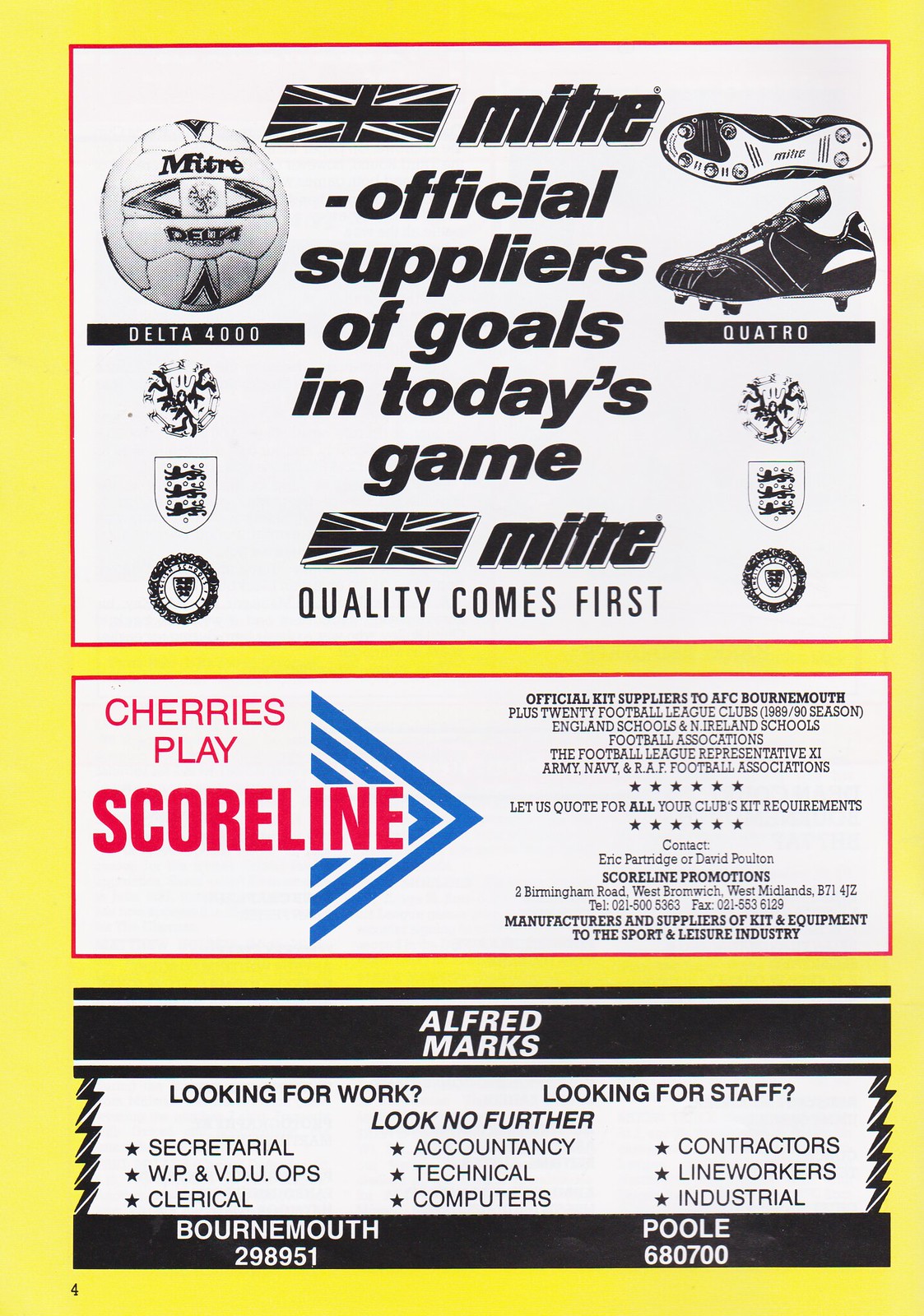The image features a yellow-background poster advertising various soccer-related services and products. At the top of the poster, a large white square with a red border showcases the soccer equipment company Mitre. It displays a black-and-white soccer ball labeled "Delta 4000" on the left and a pair of black-and-white cleats labeled "Quattro" on the right. Beneath each product are three logos. The central text reads "Official suppliers of goals in today’s game," and additional text emphasizes the brand's quality with the statement "Quality comes first."

Below this, the middle rectangular section highlights Cherry's Play Scoreline. Red text indicates "Cherry's Play" and “Scoreline” alongside blue arrows and small, unreadable black text. Cherry's Play is noted as the "Official kit suppliers to AFC Bournemouth," as well as for 20 football league clubs, Army, Navy, and RAF football associations, among others. The section includes contact information for Scoreline Promotions in West Midlands, detailing services for manufacturing and supplying sports kits and equipment.

The bottom rectangular section is an advertisement for Alfred Marks, featuring a black box with jagged edges. It offers a wide range of employment services with the phrases "Looking for work?" and "Looking for staff? Look no further." This section lists various job categories, including secretarial, clerical, technical, contractors, computers, and more. It provides contact numbers for Bournemouth (298-951) and Poole (680-700).